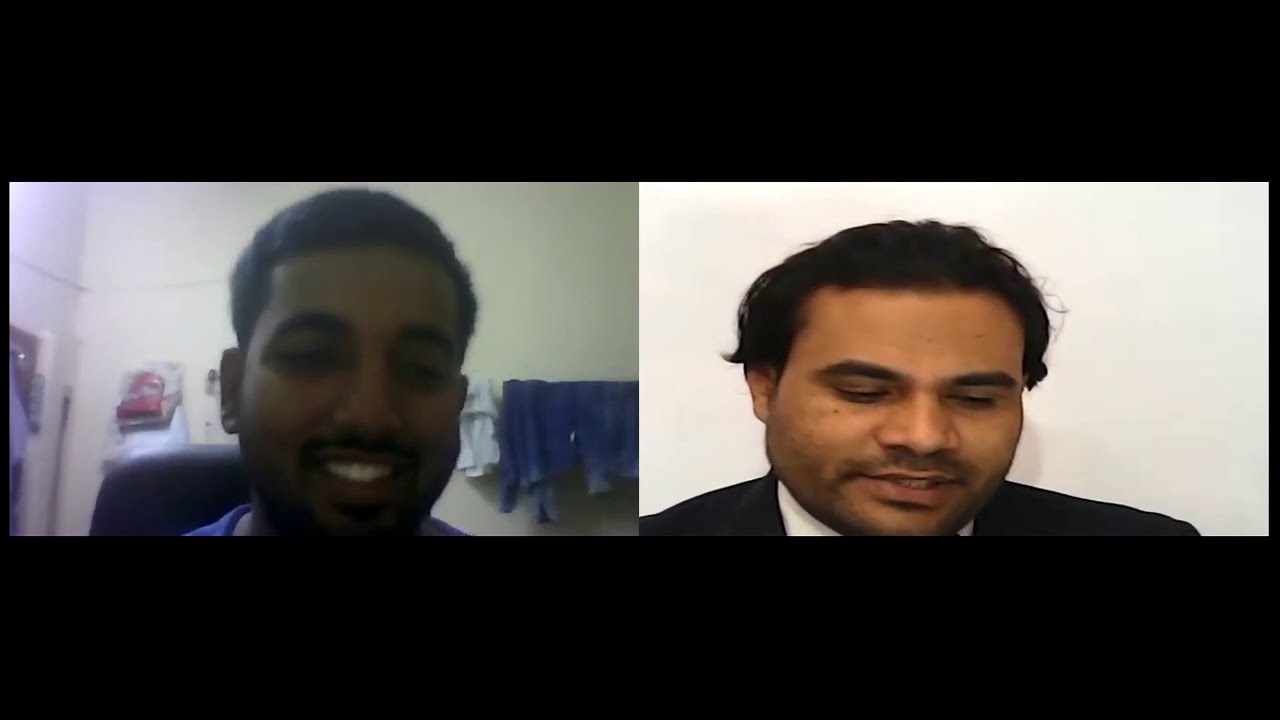The image displays a still from what appears to be a video call or a TV show, divided into two distinct sections featuring the faces of two men. On the left side, the man with short black hair and dark brown skin is seated in a chair, smiling broadly, revealing his teeth. He's wearing a blue shirt, and behind him, the white walls of his room are adorned with clothes hanging from ropes. The man on the right side also has short black hair and wears a black coat over a white shirt. He has stubble on his face and his eyes are directed downwards, giving the impression of him speaking. The background is solid white for both men. The entire composition is framed by horizontal black strips at the top and bottom of the image.